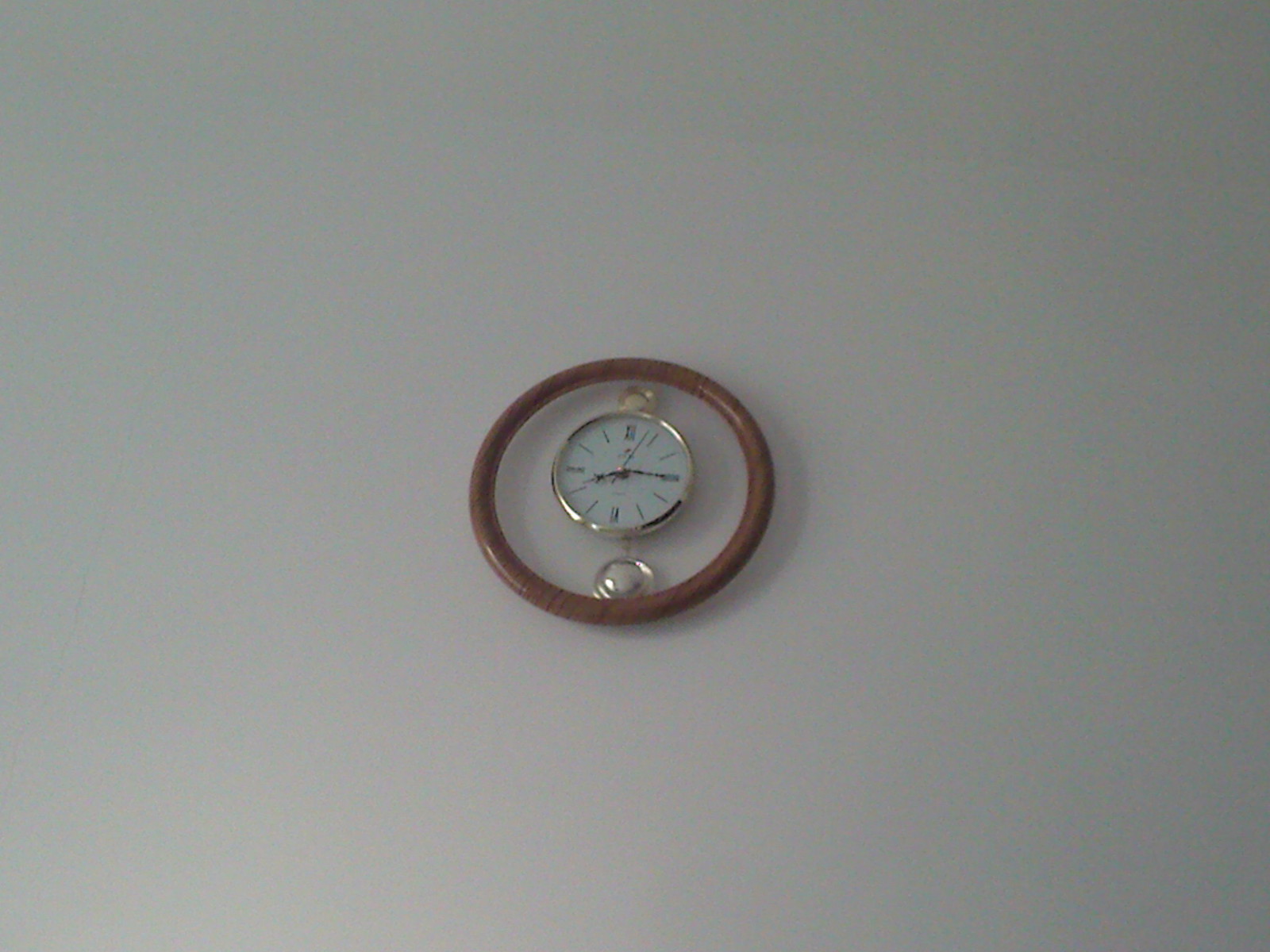The photograph showcases a unique decorative clock set against a plain, possibly grayish white backdrop. It appears to be placed on a counter rather than hanging on a wall. The clock features a medium brown wooden ring that encases the entire structure. At the very center, there is a white clock face with Roman numerals for the 12, 3, 6, and 9 positions, while the other hour markers are simple hash marks. The clock's hands for hours, minutes, and seconds are black and somewhat ornate, though the minute details are not clearly visible. Surrounding the clock face is a golden metallic rim.

Adding to the design, two small circles, one gold and one silver, are attached to the clock—one positioned above and one below. Notably, the clock is designed in an open style, allowing visibility through its various components except for the mentioned circles and frame. The time displayed on the clock is 8:15.